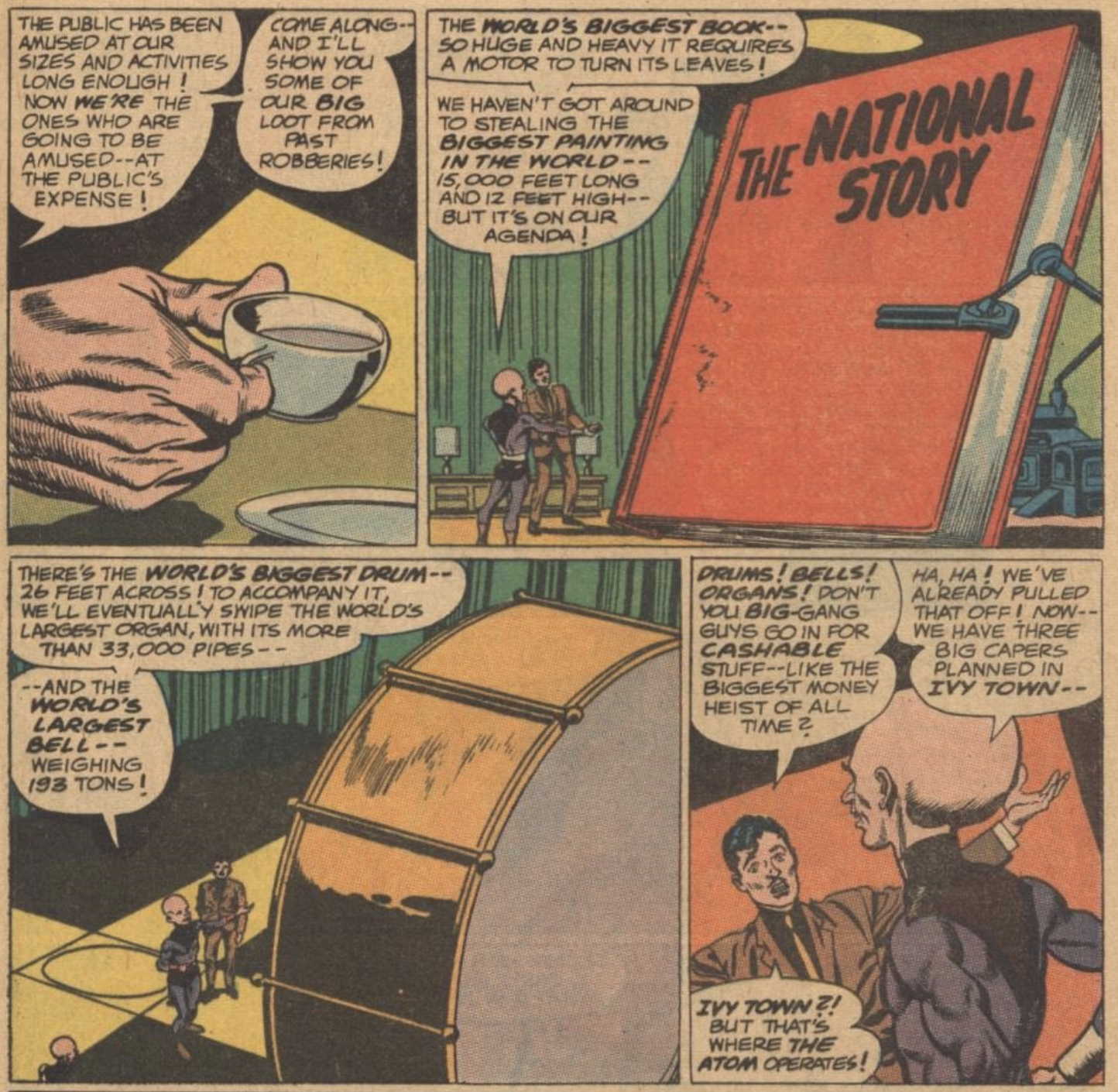This detailed caption describes a classic comic strip featuring four panels with vibrant colors including black, white, gray, green, brown, pink, blue, yellow, orange, and red. In the upper left panel, a hand delicately holds a small teacup of coffee next to a speech bubble proclaiming, "The public has been amused at our sizes and activities long enough. Now we're the ones who are going to be amused at the public's expense. Come along, and I'll show you some of our big loot from past robberies."

The next panel showcases a towering orange book titled "The National Story" in black letters, far larger than the two men standing next to it. One is a bald, large-headed figure in a bodysuit, pointing at the book and remarking, "The world's biggest book, so huge and heavy it requires a motor to turn its leaves. We haven't got around to stealing the biggest painting in the world, 15,000 feet long and 12 feet high, but it's on our agenda."

In the bottom left panel, the two men—now confirmed to be standing next to a massive drum—listen as the bald figure continues, "And yes, there's the world's biggest drum, 26 feet across. To accompany it, we'll eventually swipe the world's largest organ with its more than 33,000 pipes and the world's largest bell weighing 193 tons."

Finally, in the bottom right panel, the man in the suit questions, "Drums, bells, organs? Don't you big gangs go in for cashable stuff like the biggest money heist of all time?" The bald figure responds with a laugh, "Haha, you've already pulled that off. Now we have three big capers planned in Ivy Town," prompting the man in the suit to exclaim, "Ivy Town? But that's where the Atom operates!" This comic strip excerpt, filled with exaggerated proportions and whimsical dialogue, captures the spirit of classic comic book storytelling.